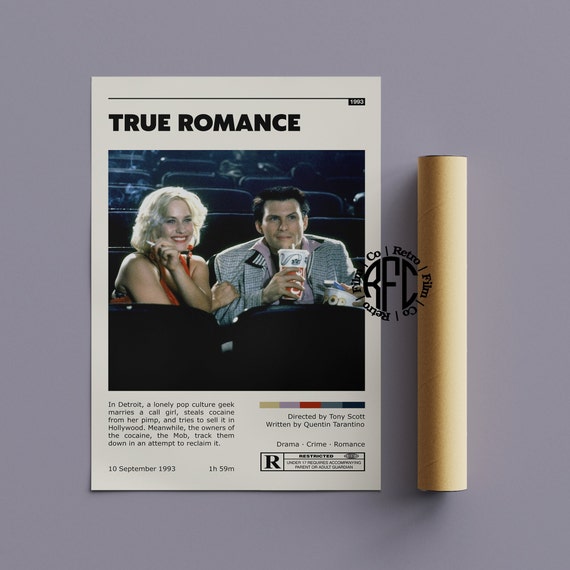The image captures a retro movie poster for the film "True Romance" set against a purplish background. Prominently displayed is a photograph of two actors sitting in a movie theater, with the male actor holding a large soda and the female actor, who has blonde hair, smoking a cigarette. Both appear to be reacting to something on the screen, the man with a hunched posture suggesting fear. The text above and below the image provides a brief synopsis: "In Detroit, a lonely pop culture geek marries a call girl, steals cocaine from her pimp, and tries to sell it in Hollywood. Meanwhile, the owners of the cocaine, the mob, track them down in an attempt to reclaim it." The film is directed by Tony Scott and written by Quentin Tarantino, falling into the drama, crime, and romance genres, and is rated R. The poster also features a watermark with the logo 'RFC,' denoting Retro Film Co., and includes the release date, September 10th, 1993, and a runtime of 99 minutes. An adjacent beige tubular container completes the composition.